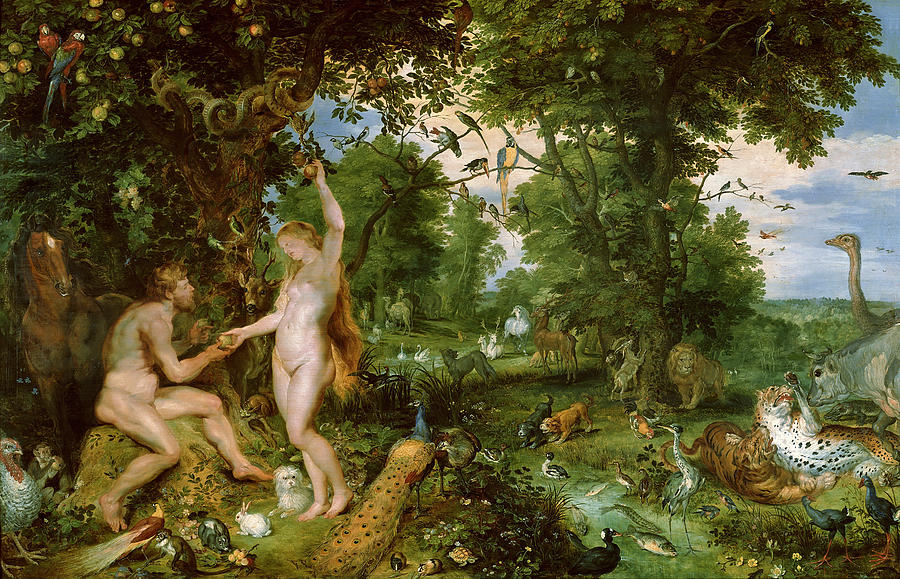This detailed digital image, evocative of a classic Garden of Eden painting, captures a vivid, intricate scene filled with a variety of animals and a Caucasian couple, Adam and Eve. The bright blue sky with scattered clouds suggests a daytime setting. The couple is positioned in the lower left-hand corner: Eve, with long, reddish-yellow hair, stands reaching up for an apple from a tree where a snake coils around the limb, while Adam sits on a stone nearby, extending his hand towards her. Both are naked, consistent with traditional portrayals.

Surrounding the couple is an array of animals from the Biblical book of Genesis. To the right of the scene are two tigers in mid-fight and a calm lion resting under a tree. Diverse fauna populate the wooded, forested area: curious parrots with red chests and blue wings plus one yellow and blue parrot, ostriches, a horse, camels, oxen, and even a distant swan swimming in a pond. Dogs, rabbits, and deer are also present among the dense vegetation, adding to the richness of the scene. Floating in the sky among various birds, there's an unusual sight — what appears to be an airplane, contrasting with the traditional elements of the artwork.